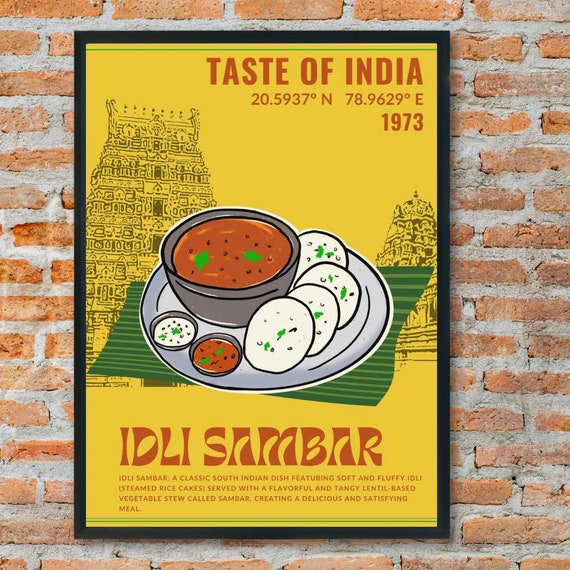This framed picture, set in a sleek black frame against a red-orange brick wall with heavy mortar, showcases a vibrant yellow poster entitled "Taste of India" in bold red letters. Below the title, the latitudinal and longitudinal coordinates 20.59° N, 78.96° E and the date 1973 are displayed, pinpointing a specific location in India. Central to the poster is an intricate drawing of a traditional South Indian meal. It features a plate containing four neatly sliced pieces resembling cucumber, flanked by two small containers of contrasting red and white sauces. At the heart of the plate is a small bowl filled with a rich brown liquid, all resting on what appears to be a green tablecloth.

The background of the poster includes a sketch of a distinctively Indian six or seven-story building, adding cultural context. At the bottom, "Idli Sambar" is inscribed in brown letters against the yellow canvas. Beneath this title, in fine print, the text reads: "Idli Sambar, a classic South Indian dish featuring soft and fluffy steamed rice cakes served with a flavorful and tangy lentil-based vegetable stew called Sambar, creating a delicious and satisfying meal." The detailed description rounds off the overall presentation, merging visual and textual elements to celebrate the culinary heritage of South India.